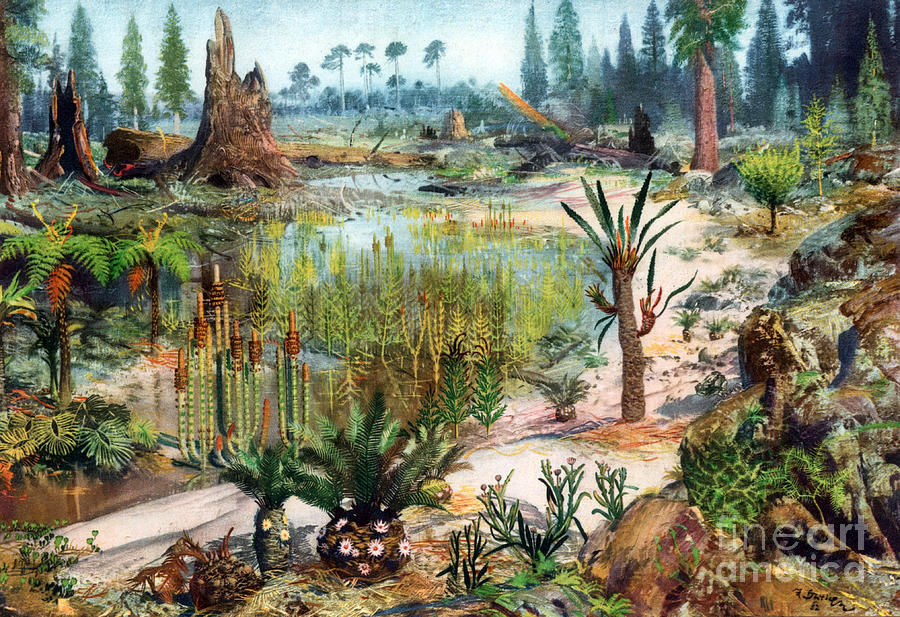This color painting, in landscape format, presents an impressionistic depiction of a lush, marshy forest landscape filled with diverse vegetation, giving it a prehistoric atmosphere. The foreground features small pine trees, varied vegetation including ferns and flowering cacti, as well as moss-covered rocks in shades of brown and gray. The right-hand side shows a protrusion of boulders, while the lower right corner is stamped with "Fine Art America" in white letters.

Moving deeper into the scene, low scrubby plants mix with a few patches of white dirt and a small water area filled with rushes. On the left, an enormous broken tree trunk lies on the ground next to a large stump, while another immense felled trunk lies in the middle, resting across the stream. The background is densely packed with a variety of trees, including tall palm-shaped and cypress-like trees, that enhance the prehistoric feel of the scene. The sky overhead is a blend of grayish blue tones with some lighter patches, completing the natural and untouched ambiance of the painting.